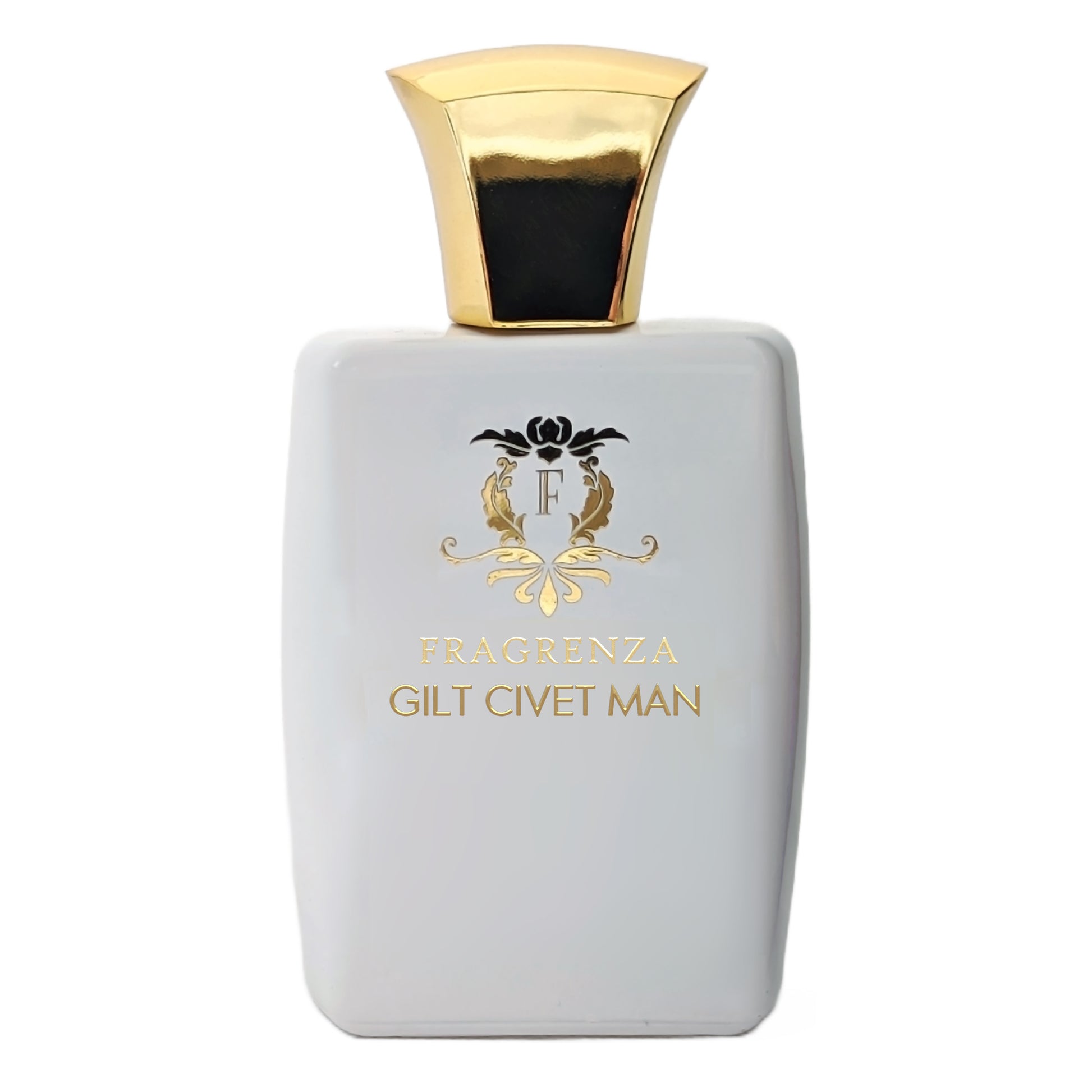The image depicts a white rectangular bottle, likely of cologne, set against a clear black backdrop. The bottle features an ornate, square-shaped gold cap that flares out before tapering at the top. It is adorned with an intricate crest pattern consisting of filigree elements such as leaves and scrolls. At the center of this crest is an embossed gold letter "F," and just below it, the word "FRAGRENZA" is elegantly inscribed. Beneath this, the label reads "GILT CIVETTE MAN," indicating it is a product for men. The overall design and gold accents give the bottle a luxurious and potentially high-end appeal.